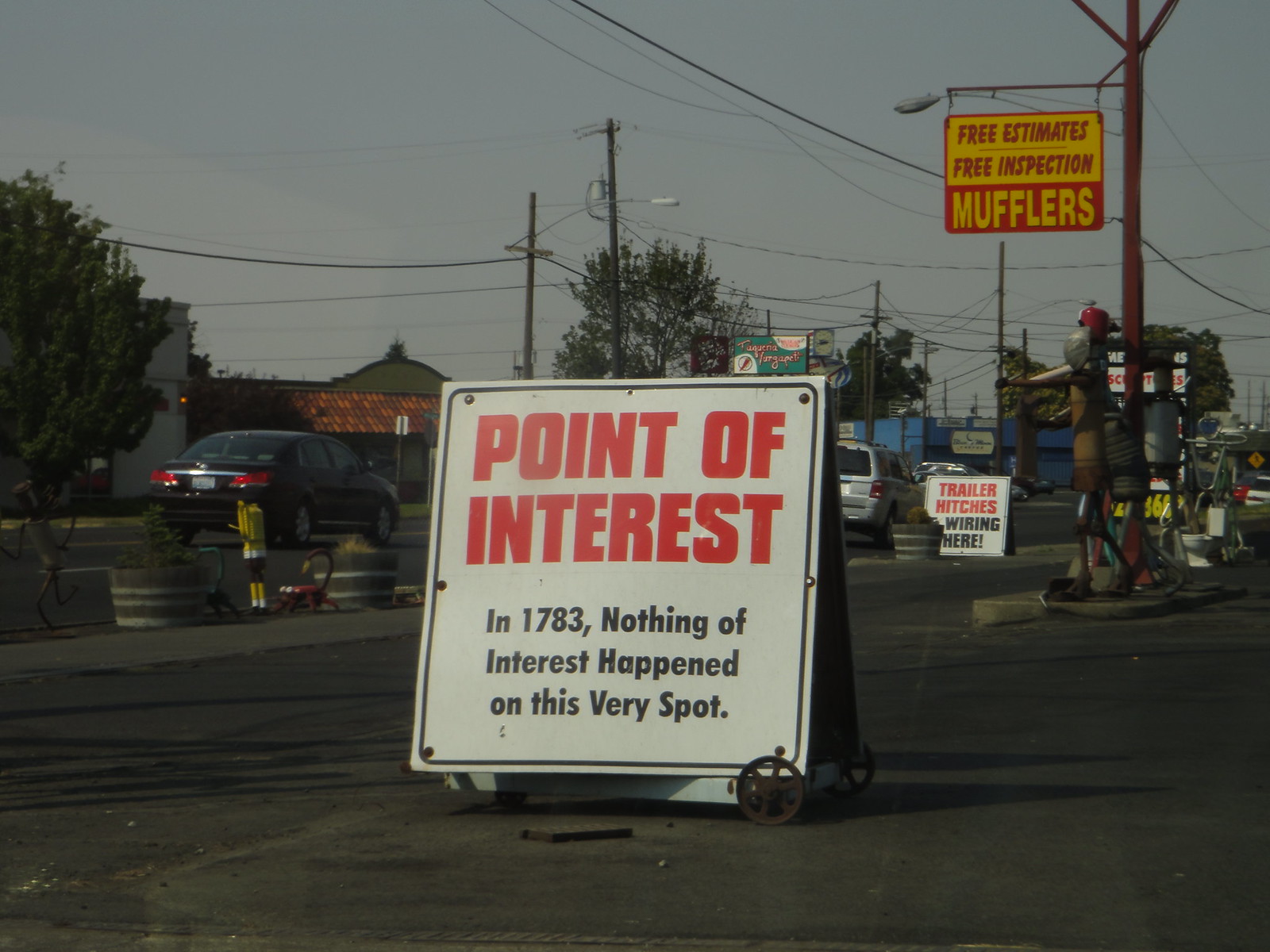The image captures an outdoor scene under a dim, blue-gray foggy sky. Dominating the center is a large white sign with a black border. This sign reads in bold red letters, "Point of Interest," and below in smaller black font, "In 1783, nothing of interest happened on this very spot." The sign is mounted on gray concrete. Behind it, there's a bustling scene with various cars driving down the street, including a black sedan and a gray SUV. A light pole in the background features a red and yellow sign advertising, "Free Estimates, Free Inspection, Mufflers," with the mufflers portion displayed in yellow letters on a red background. Nearby, another sign reads, "Trailer Hitches, wiring here." A metal sculpture, possibly resembling a person, stands at the base of the light pole. The backdrop includes several buildings, numerous electrical poles, and scattered trees, contributing to the busy urban setting.